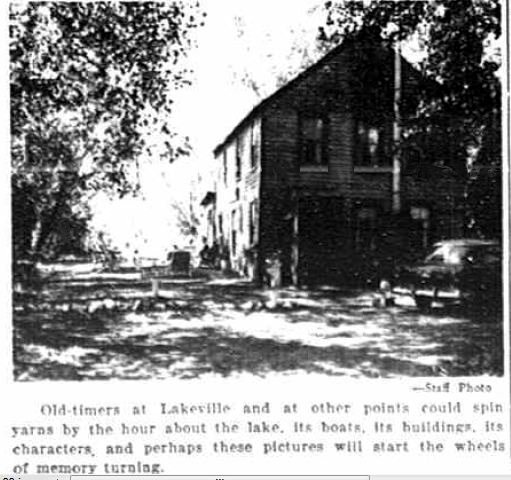A vintage and blurry black-and-white photograph, likely a printed newspaper clipping, depicts an old two-story wooden house set in a wooded area. The house is large and viewed from the side, with trees in the foreground. Parked in front of the house is a classic 1950s Chevy-looking car, adding to the nostalgic feel of the image. On the left side of the photograph, some people can be seen sitting perhaps on lawn furniture or a small deck, though the details are hard to discern due to the poor quality. The photograph is accompanied by a caption at the bottom that reads, "Old-timers at Lakeville and at other points could spin yarns by the hour about the lake, its boats, its buildings, its characters, and perhaps these pictures will start the wheels of memory turning." The overall image is part of a printed vintage publication, characterized by its realism and historical charm.